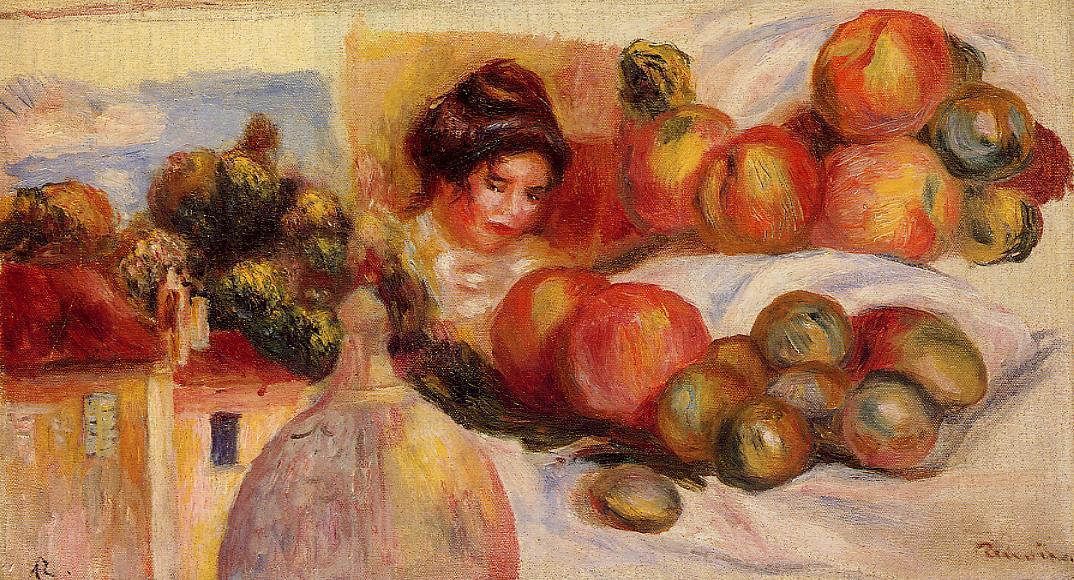The image depicts a hand-painted post-impressionist artwork, characterized by warm, orangey tones. Central to the composition is the sad, closed-eyed face of a woman with dark hair styled in an early 20th-century bun, wearing what appears to be a light-colored or pale pink top. Her face and head are positioned directly in the center of the painting. Surrounding her are various fruits, likely oranges or peaches, arranged in clusters, some of which are resting next to a large vase or urn in the bottom left. The right side of the painting prominently features these fruits as well. To the left, there are buildings with trees on the roof, and above them, a blue sky with clouds is visible, adding depth to the scene. The painter meticulously balanced the elements in the artwork, ensuring an evenly spaced and harmonious layout. The artist's signature, likely "Renoir," appears in brown in the lower right corner, reinforcing the painting's authenticity and craftsmanship.